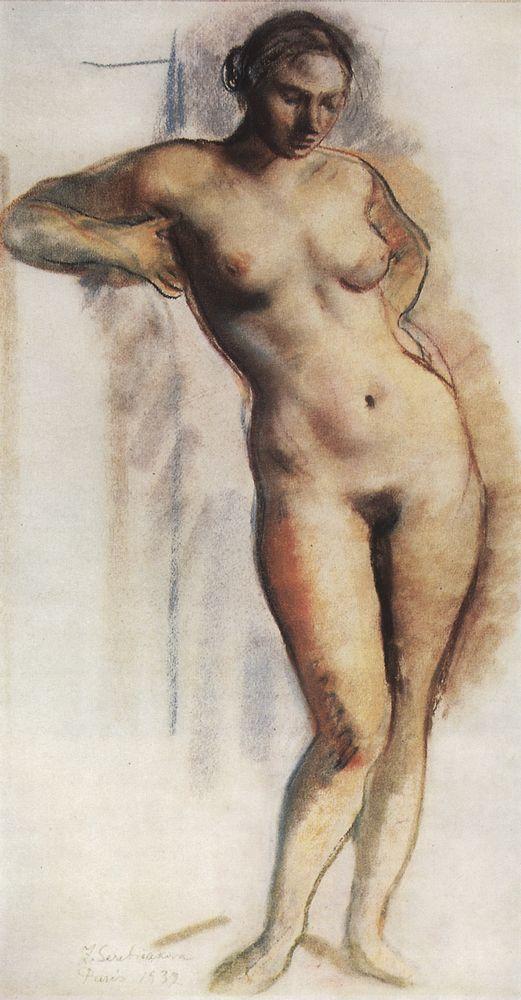This detailed charcoal drawing or painting portrays a nude woman standing against a primarily white wall with minimal background details, lending the focus to her form. The artwork meticulously captures the anatomy of her breasts, belly, and thighs, while lesser emphasis is placed on her hands, arms, legs, and feet. The woman stands looking downward, her striking black hair tied back. Her right arm is extended almost straight, with her elbow leaning against the wall and her thumb touching her armpit. Her left hand rests on her hip. Her beautifully rendered face, while somewhat realistic, is shadowed on one side, with her eyes seemingly closed. The artwork uses skin tones, browns, whites, and grays, with significant shading to enhance the realism of her figure, which includes visible details such as her nipples, navel, pubic area, and curvaceous form.